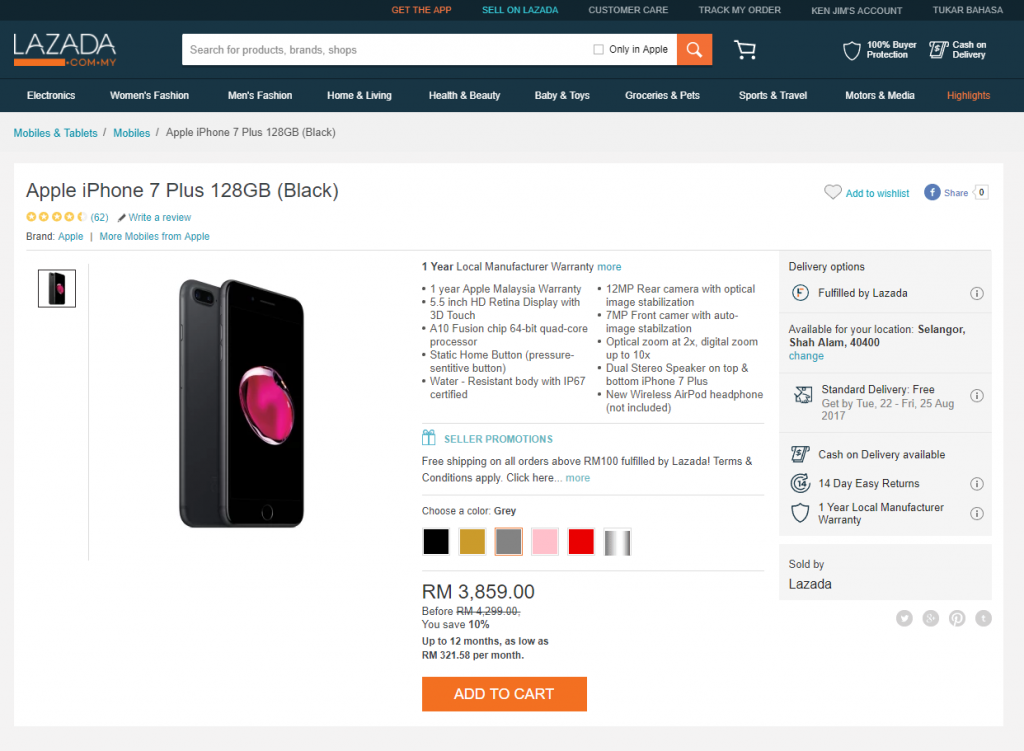Detailed Caption for Lazada.com.my Screenshot:

The screenshot captures the Lazada.com.my website interface. The top section features a black background with key navigational elements. In capital orange letters, the text "GET THE APP" is prominently displayed. To its right, the blue text "Sell on Lazada" is followed by links for "Customer Care," "Track My Order," "Ken Jim's Account," and "Tukar Bahasa."

Below this top strip is the Lazada logo in dark blue lettering, accompanied by a search bar for products, brands, or shops, and a shopping cart icon. A message stating "100% Buyer Protection" is also visible, providing assurance to potential buyers.

The main content area of the screenshot highlights a product listing for an Apple iPhone 7 in black with 128 GB of storage. The image of the iPhone features a clear digital display. Detailed specifications of the phone are outlined, including information about the seller, delivery fee, returns, and warranty policies. The listed price is RM 3859, with an option for the user to select the color of the phone.

Overall, the screenshot provides a comprehensive overview of the Lazada website's layout and a specific product listing.